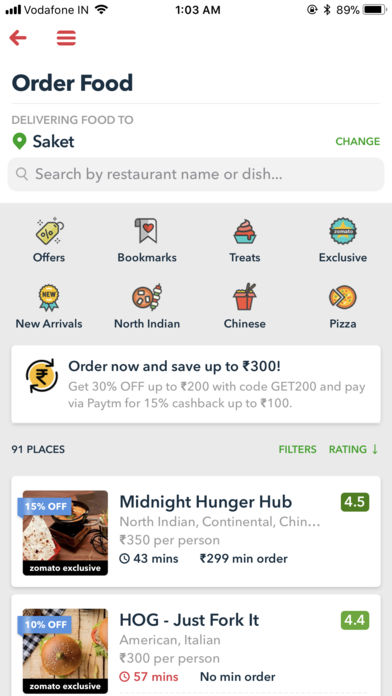The image is a screenshot from a smartphone, featuring a predominantly white background. At the very top left corner, there's an icon indicating the wireless connection, labeled "Avoda Phone IM," which is the wireless carrier. To the right of this, the Wi-Fi icon is visible. Centered at the top is the time, displayed as 1:03 a.m. On the upper right corner, a battery icon shows a charge level of 89%.

Beneath the "Avoda Phone" label on the left side, there are three small horizontal red lines, indicating a menu. To the left of these lines is a red arrow. Below this section, bold text reads "Order Food," followed by the phrase "Delivering Food To" in gray font, accompanied by a green location marker icon next to the name "SAKET," presumably the location or city.

Below this, a long rectangular gray search bar is present. Further down, there's a gray box featuring cartoonish images labeled with categories like offers, bookmarks, treats, exclusive, new arrivals, North Indian, Chinese, and pizza.

A white rectangular section follows with a headline in dark gray text that reads, "Order Now and save up to 300," though the currency is unspecified. Below this promotional message, two restaurant listings appear, each within its own white rectangular box. The first restaurant, "Midnight Hunger Hub," has a rating of 4.5 displayed in a green square. The second restaurant, "HOG Just Fork It," boasts a rating of 4.4.